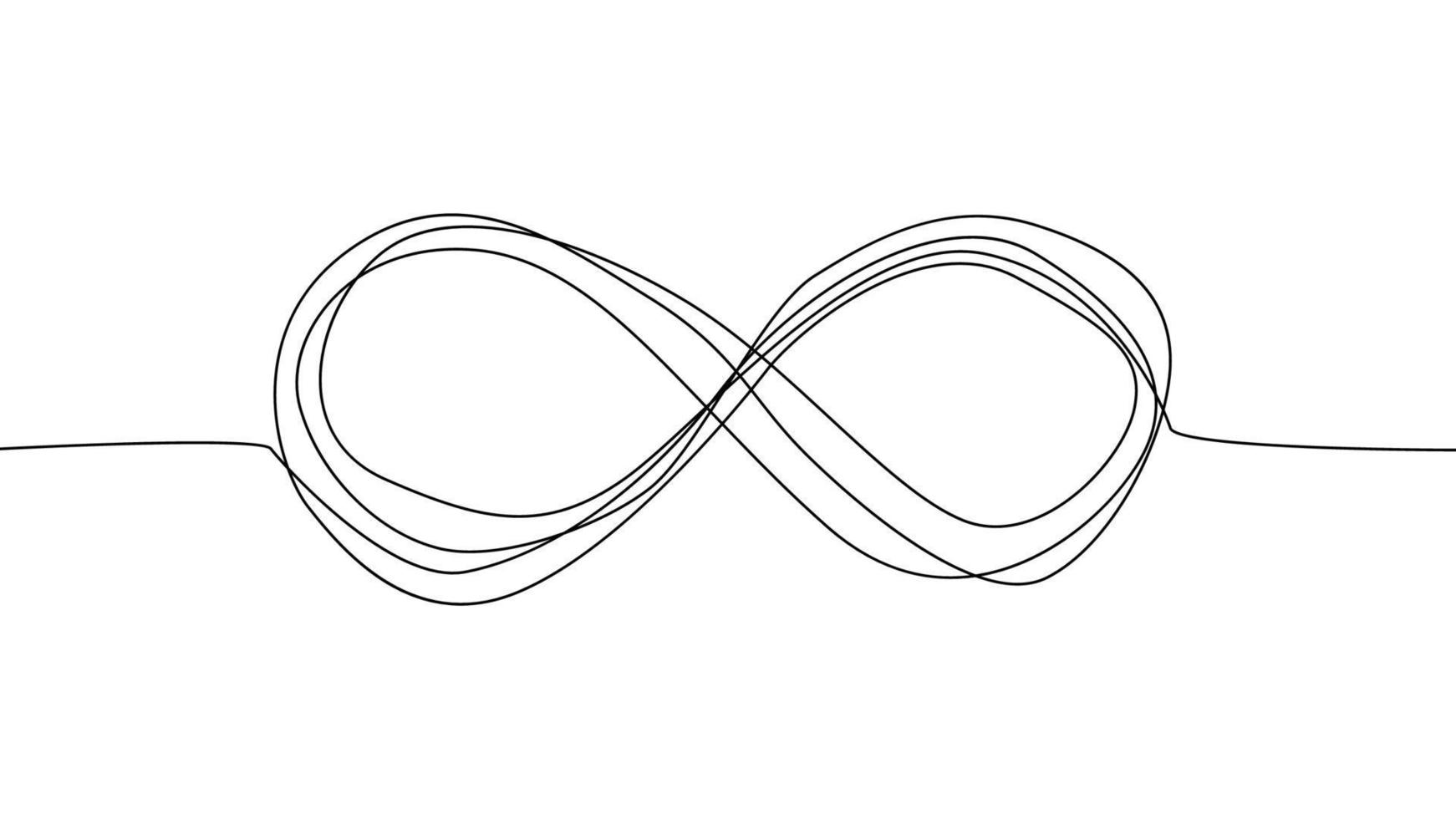The image appears to be a digitally generated drawing consisting of two overlapping, rough infinity signs, created with black lines against a white background. The lines loop around multiple times, resembling a black thread with ends on both the left and right sides. The loops intersect in the middle, forming a complex figure-eight shape that has been traced several times. The overall impression is akin to a child's doodle or a playful sketch that could also be seen as a pair of designer glasses or a racetrack, but the lines lack precision, adding to its abstract and whimsical appearance.